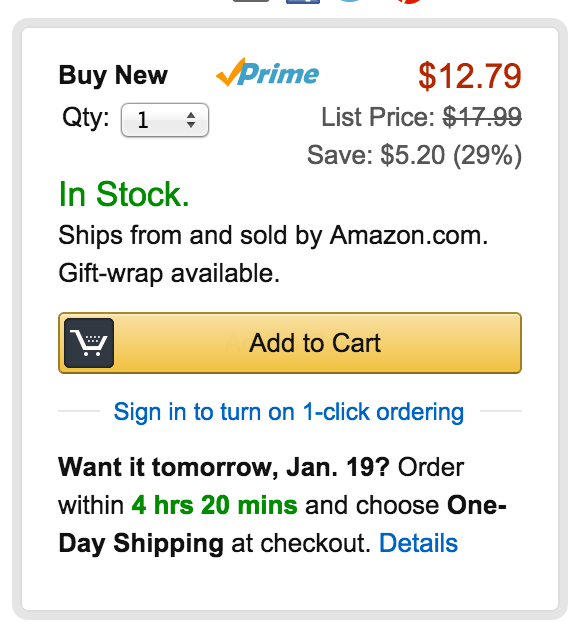This is a detailed screenshot of a pop-up menu on Amazon.com. The menu is bordered with gray lines and has a white, square-shaped center. In the top left corner, in bold black font, it says "Buy New." To the right, there's a yellow checkmark accompanied by blue text that reads "Prime." Further to the right, in red font, is a dollar sign followed by the price "$12.79."

Directly below, on the left side, it says "QTY:" followed by a gray rectangular drop-down menu displaying the number "1." Adjacent to this, in dark gray font, it says "List Price: $17.99," with a strikethrough line indicating a discount. Below, it states "Save: $5.20 (29%)."

In red font, it indicates "In Stock." Below this, in black font, it mentions "Ships From and Sold By Amazon.com" and "Gift Wrap Available." At the bottom, there's an orange rectangle featuring a cart icon on the right side, symbolizing the option to add the item to the shopping cart.